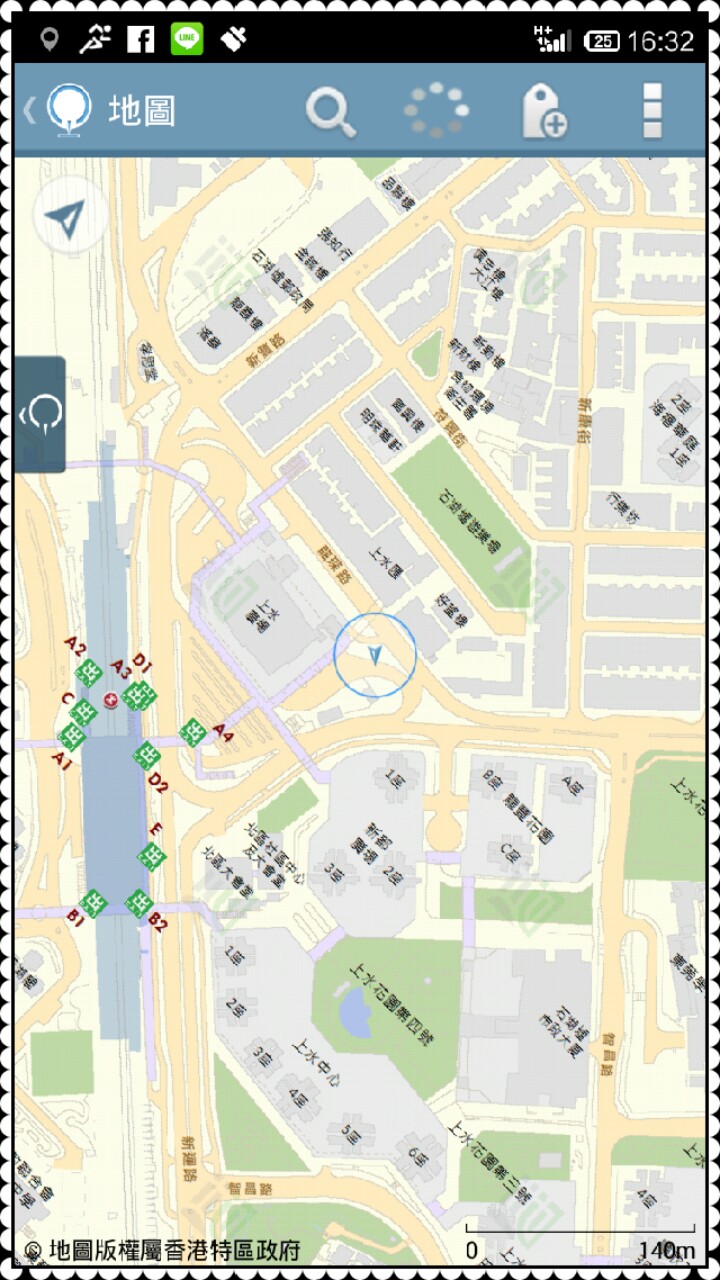The image depicts the top portion of a screen featuring a black bar filled with various icons. From left to right, the icons include a lightbulb, a running person, a white square with a black 'F', a green square containing a speech bubble, a paintbrush, a signal strength icon showing four out of five bars, and a battery icon displaying '25' with '16:32' written next to it.

Following these icons are a blue rectangle with a left-facing arrow, a circle within another circle, an Asian character which is likely Chinese, a magnifying glass, a loading symbol, a tag icon resembling a square with a circle at the top, a plus sign in the bottom right corner, and a vertical stack of three squares.

The center of the image shows a navigation map, likely depicting an area in China, characterized by intersecting rows of buildings in gray, green, and yellow. A watermark is visible, though it is not clearly identifiable. In the bottom left corner, there is more information presented in Chinese characters, along with a scale ranging from 0 to 140 millimeters.